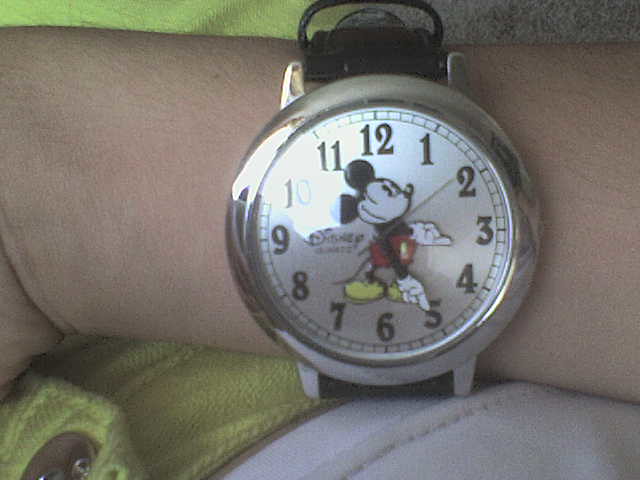This close-up image captures a classic Mickey Mouse wristwatch, securely fastened on the inner wrist of a person with a light skin tone and faint arm hairs. The wrist is angled across the person's stomach, over a yellow and white fabric that appears to be their blue jeans and short sleeve white t-shirt. The round watch face, encased in a chrome-like metal body, prominently displays Mickey Mouse at the center. Mickey is attired in his iconic red shorts with yellow buttons, white gloves, and yellow shoes, and he looks to the right. His gloved hands serve as the hour and minute hands, pointing to 3:25, while a thin second hand points towards the number 2. The background is silver, and each black number is clearly visible around the watch face. The word "Disney" is inscribed in black cursive to Mickey's left. The black watch band, likely made of a soft leather material, is partially visible at the top of the photo. A distinct reflection of light can be seen between the 10 and 11 on the watch face, adding a glint to this charming timepiece.